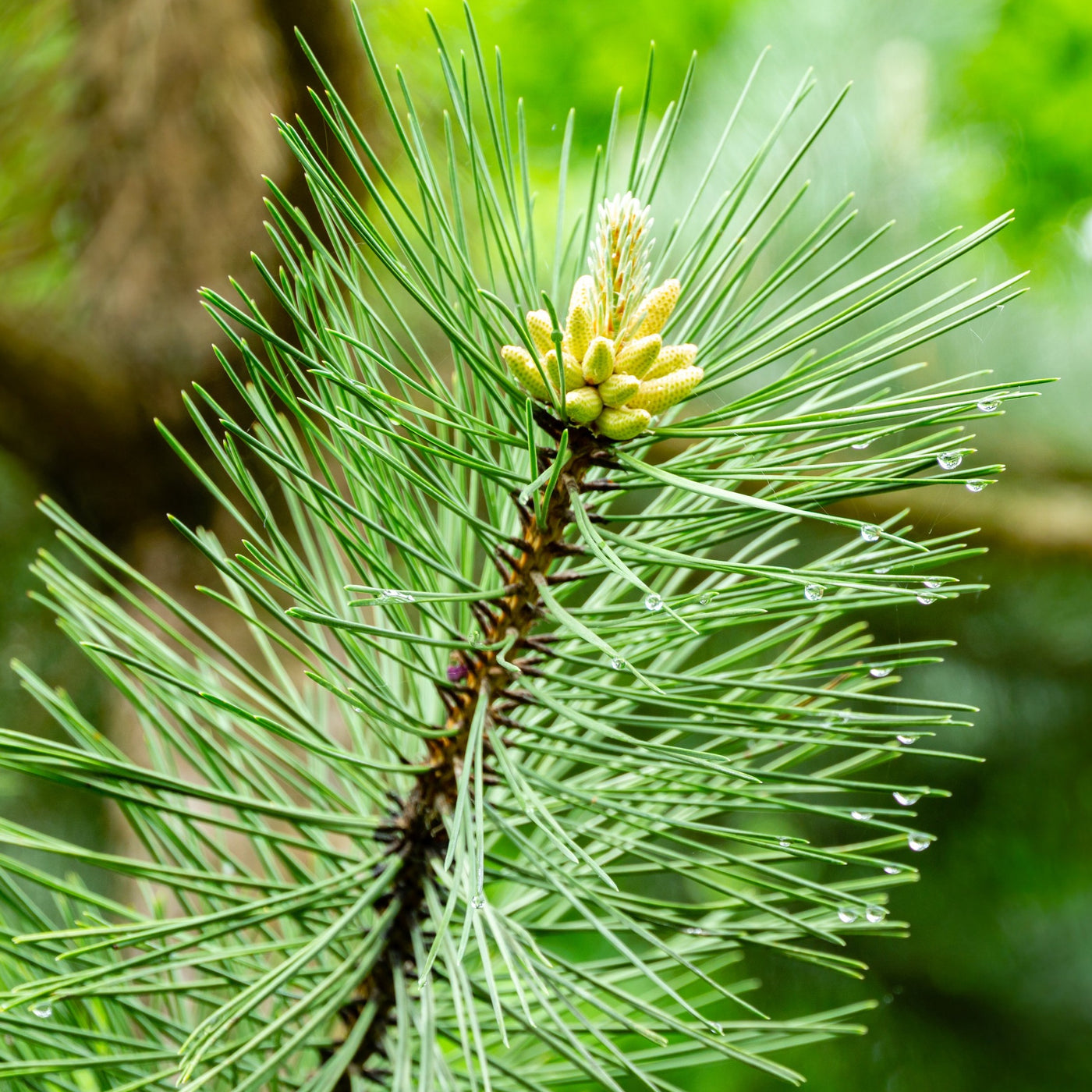The image is a close-up of a slender dark brown branch from a pine tree, featuring numerous long, light green needles protruding symmetrically on both sides. Distinctively, several of these needles on the right side of the branch are adorned with tiny water droplets, suggesting recent rain or a moist environment. At the top of the branch, there are several yellow, corn-like formations that resemble flowering buds. The photo captures the intricate details of the pine while the background remains blurry, filled with varied green hues and some brown areas, indicative of a dense forest or wooded setting.